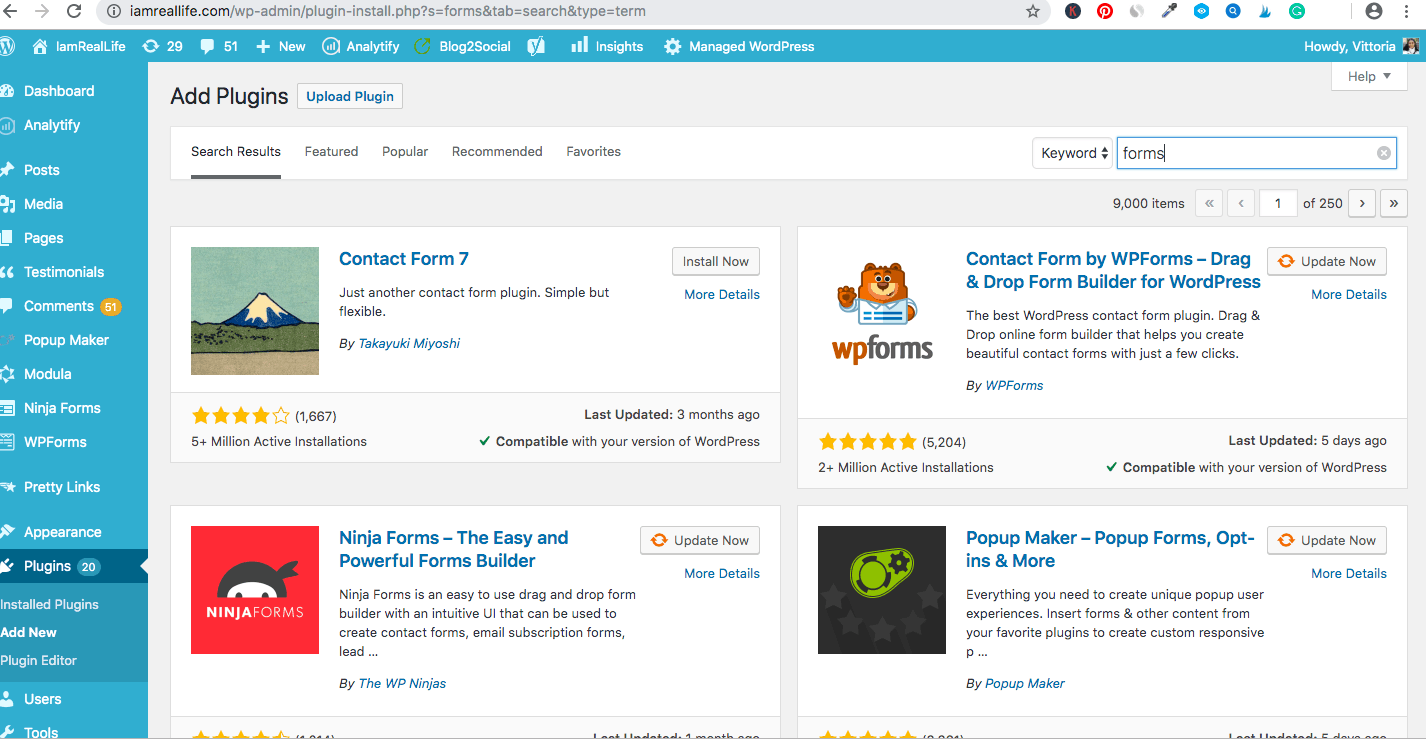On the webpage of "iamreallife.com," we are viewing a section titled "Add to Plugins." This interface displays various plugin modules, each accompanied by illustrative images and brief descriptions. Among the plugins featured are "Ninja Forms," described as an easy and powerful form builder, represented by a cartoon ninja icon, and "WP Forms," labeled as a contact form plugin. Each plugin appears to be a tool that can be added to enhance website functionality. 

The page layout includes a light blue toolbar at the top and a similarly colored navigation area on the left side. Another listed plugin is "Pop-Up Maker," which features an image of a gear icon. There is a search field showing that the term "forms" was used, leading to numerous form-related plugin results. Some plugins have an "Update Now" status indicating they are already installed and need updating, while others have an "Install" option suggesting they are yet to be added to the system.